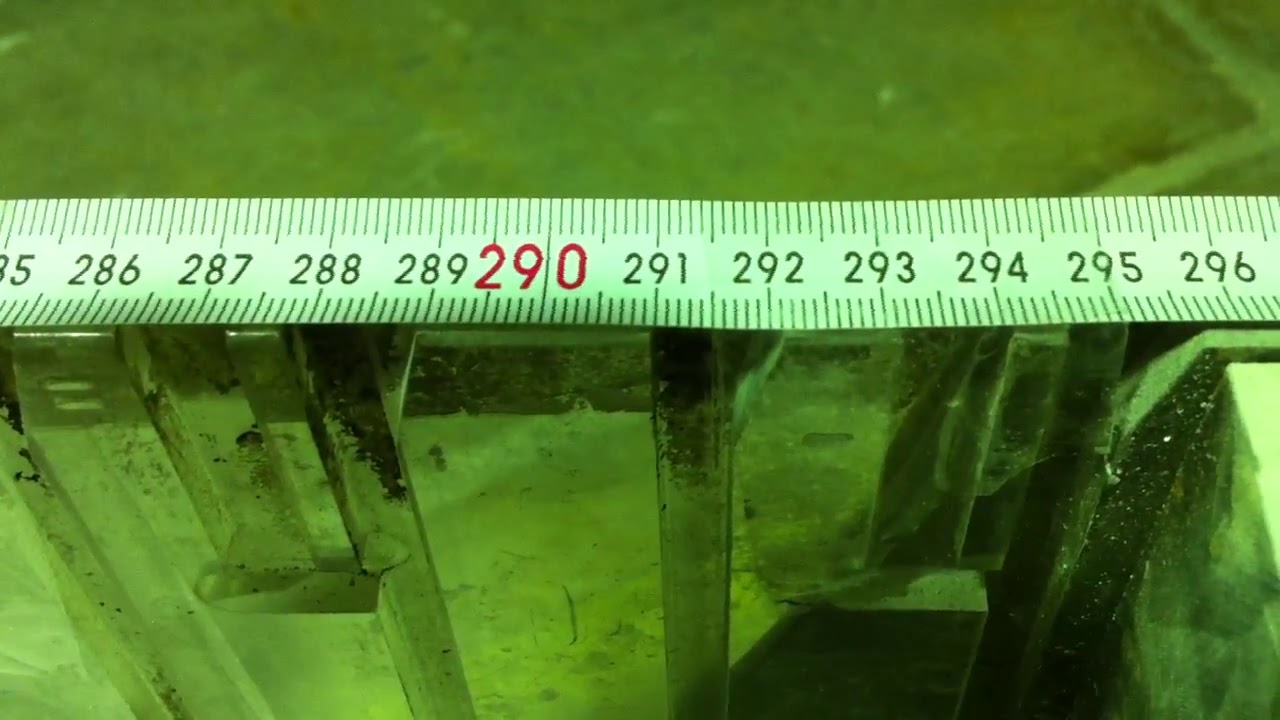The image features a horizontally aligned ruler, prominently placed across the center, measuring in centimeters. The photo is in a 16-by-9 aspect ratio, with a putrid green tint covering the entire scene. The tape measure itself is white, with black numbers and markings. Notable measurements displayed include large black numbers '290' slightly left of center, flanked by smaller black numbers from '285' (partially cut off) to '296' in the rightward direction. Beneath the ruler, there appears to be a metallic, reflective flat surface that may resemble a rail guard or handlebar, which captures some indistinct black reflections. The lower half of the image shows what looks like a crystal-like structure or mechanical siding, adding to the scientific or industrial ambiance. The background is less reflective, with a darker, possibly brownish or grayish ground.